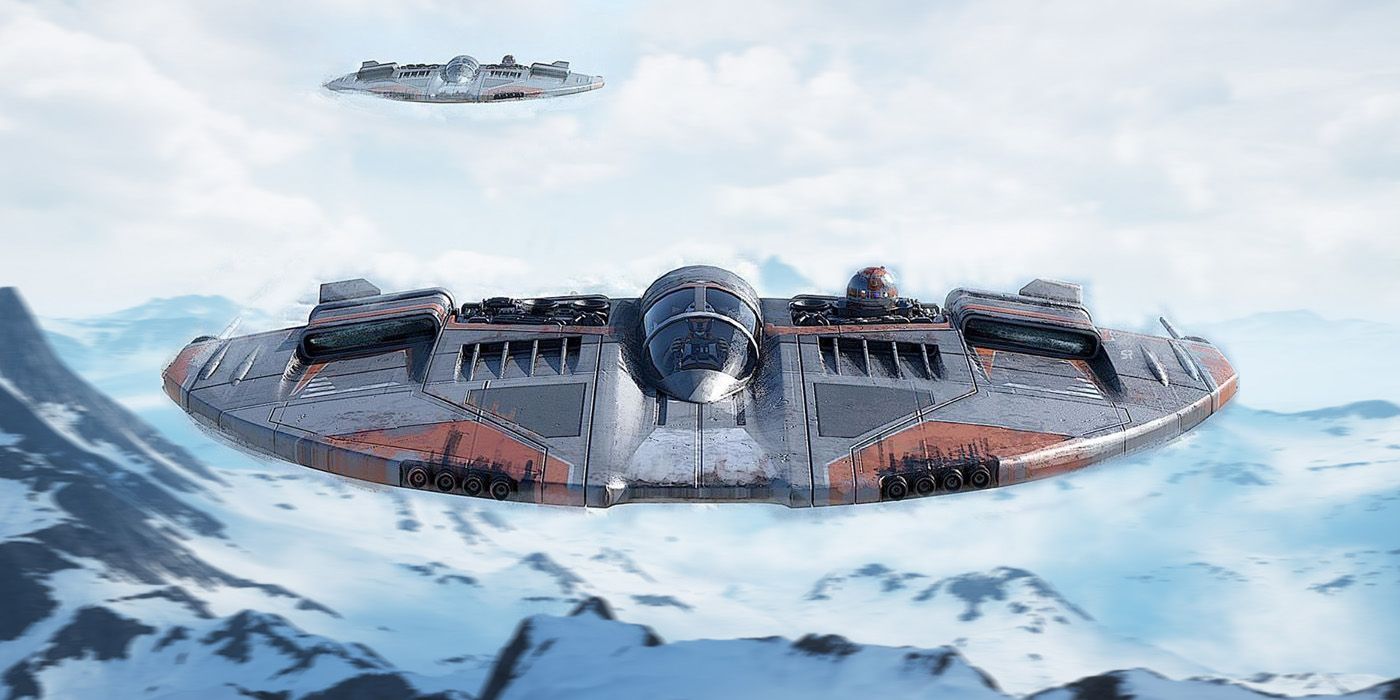The image depicts two semi-circular Star Wars ships flying over a snowy, mountainous landscape. The primary ship is prominently positioned in the foreground, facing the front, while a similar, slightly more silver-colored ship hovers in the background. The sky is overcast with white clouds, setting a dramatic scene. The ships feature a bullet-like chamber with a large, tubular glass window in the center, through which a pilot is visible. Both ships are equipped with rectangular engines on their sides and exhaust vents, with light red trim details and four small circular holes, possibly lights or guns, on the front. The landscape below is rugged and rocky, with dark brown exposed rocks covered in a blanket of snow, emphasizing the harsh, wintry environment.